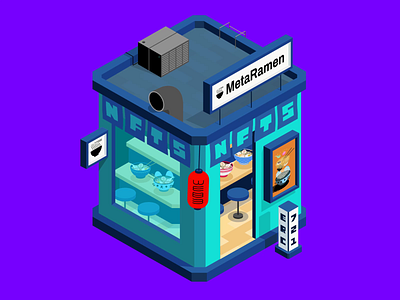The image is a vividly colored digital artwork set against a bright purple background. At the center, there is a small, square building featuring aqua blue walls. Atop the building, a rectangular white marquee prominently displays the name "METARAMAN" in bold, black letters. 

The roof of the building hosts a square-shaped furnace or air conditioning unit, accompanied by a gray cylinder that extends upward before curving outward over the edge of the roof. 

Through the windows, the interior reveals a yellow counter paired with blue stools. Resting on the counter are several bowls of food, suggesting a dining or café setting. The exterior of the building is adorned with an illustration depicting a bowl with chopsticks and a variety of food, hinting at the type of cuisine served within.